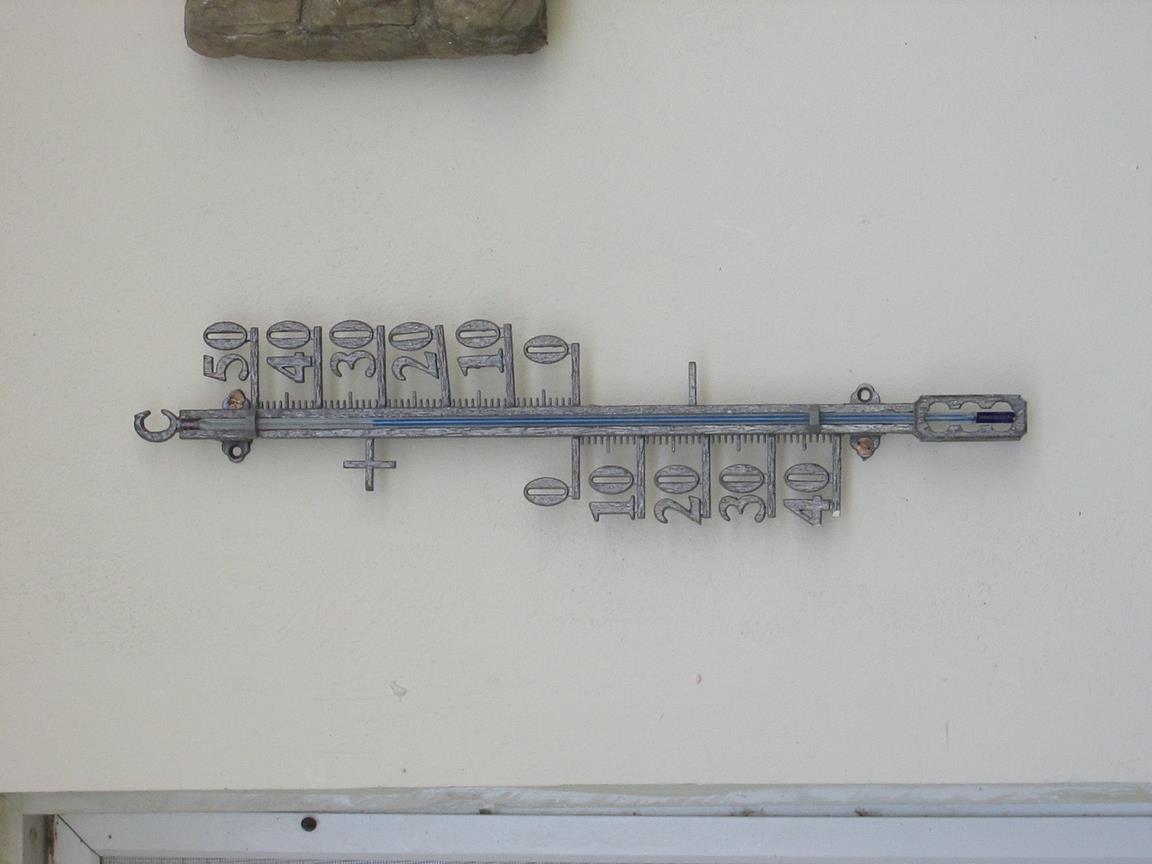This photograph showcases a vintage outdoor thermometer that exudes an old-world charm. The thermometer is crafted from what appears to be pewter, lending it a classic metallic sheen. Encased within glass, the temperature is gauged by a mesmerizing blue liquid. The thermometer’s scale is elegantly arranged with negative numbers on the left side and positive numbers on the right, each denoted by their respective negative and positive signs. The temperature readings start at the bottom from -40°C, ascending through -30°C, -20°C, -10°C, 0°C, and rise to 10°C, 20°C, 30°C, 40°C, and finally 50°C at the top. At the pinnacle of the thermometer is a prominent 'C,' indicating that the measurements are in Celsius. It is mounted securely on a pristine white wall, which captures a sense of simplicity and cleanliness. Just peeking in on the left side is a narrow frame of what may be a window or door, also in white. To the right side of the thermometer, there hangs a mysterious plaque or object constructed from gray brick, adding an intriguing touch to the composition of the wall.